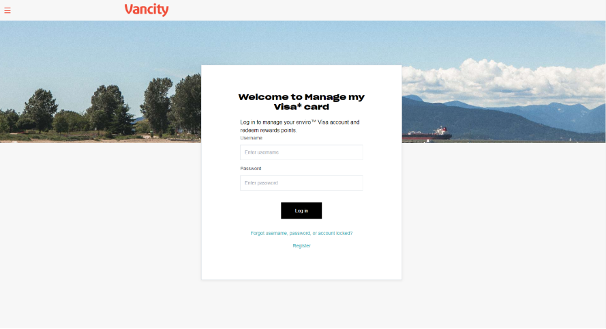The screenshot displays a webpage from a site named "Vansity," identified by its distinct orange font logo situated at the upper left corner. Dominating the background is a scenic panoramic photograph depicting an outdoor landscape. The left side of the image features lush trees, while the right side showcases majestic mountaintops partially veiled by cloud cover.

Central to the screen is a prominent white rectangle overlay that spans approximately the middle two-thirds of the image vertically. Within this white overlay, clear and bold black text reads: "Welcome to Manage My Visa Card." Below this header, the text begins to blur, making it difficult to decipher, but mention of logging in to manage your Visa card can be discerned.

The login section features input fields for a username and password. Adjacent to these fields is a black button labeled with the call-to-action: "Log in." Directly beneath this, a link is provided for users who have forgotten their username. The overall layout and design aim to blend user interface elements with a visually appealing outdoor theme.